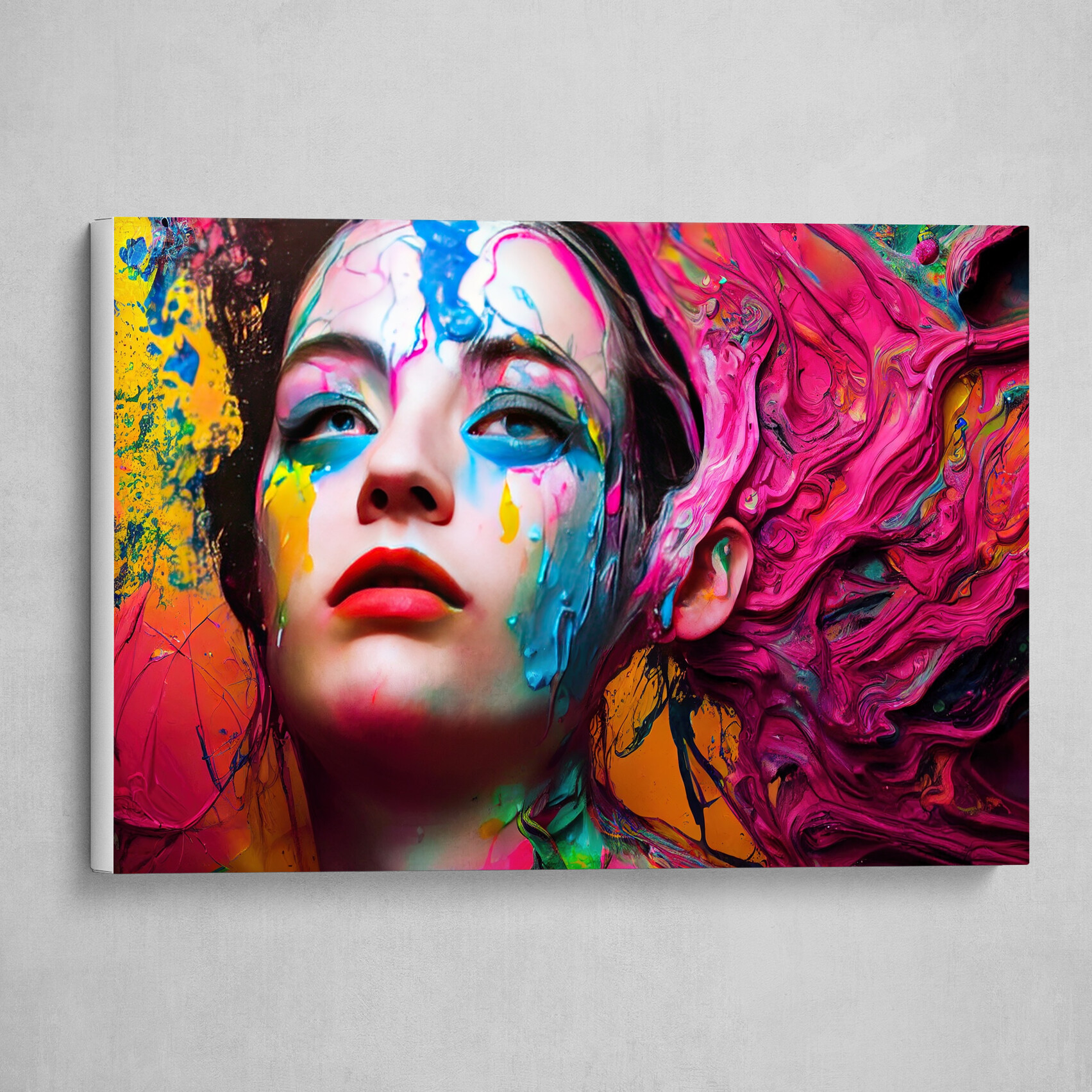Set against a square gray background, the horizontally oriented canvas depicts an intricate and colorful portrayal of a woman's face and neck, covered with a vibrant array of paint splatters. The artwork, which displays noticeable textures indicative of traditional painting techniques, primarily focuses on the woman's face adorned with various hues—yellow on her left cheek, blue around her eyes and from her forehead, and pink drips scattered across. Her red lipstick, defined eyeliner, and brownish hair that melds into the splattered colors around her, lend a strikingly realistic quality to the piece. The right side of the painting is dominated by vivid pinks, while the left side features more yellow, orange, and green tones, all blending into a dynamic, textured background. The artwork's modern and abstract composition creates a visually engaging piece that seems both animated and potentially AI-generated, blurring the lines between digital and traditional artistry.